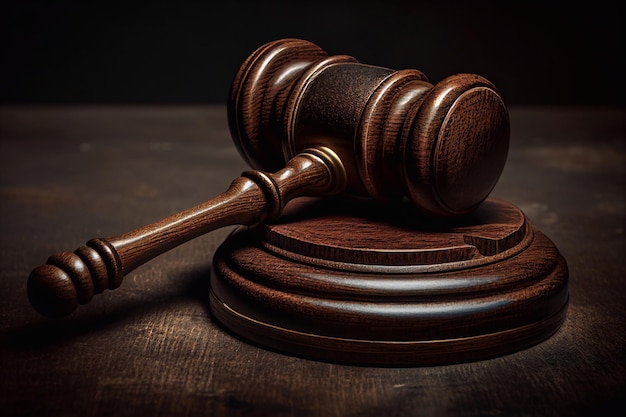This highly detailed photograph captures a sturdy, dark brown wooden gavel, similar to those used by judges in courtrooms, placed on a matching round wooden sounding block. The cylindrical head and thinner handle of the gavel are prominently featured, with the gavel itself lying on its side and the top part subtly lit by a light source from the top and right. The round sounding block, also wooden and dark brown, displays a shiny finish with a notable reflection of white light on its front. Both gavel and sounding block rest on a dark brown wooden table, which appears slightly paler as it extends into the distance. The photograph, oriented horizontally and approximately one and a half times as wide as it is tall, has a solid black background occupying the top portion, adding contrast and focus to the wooden elements central to the image.